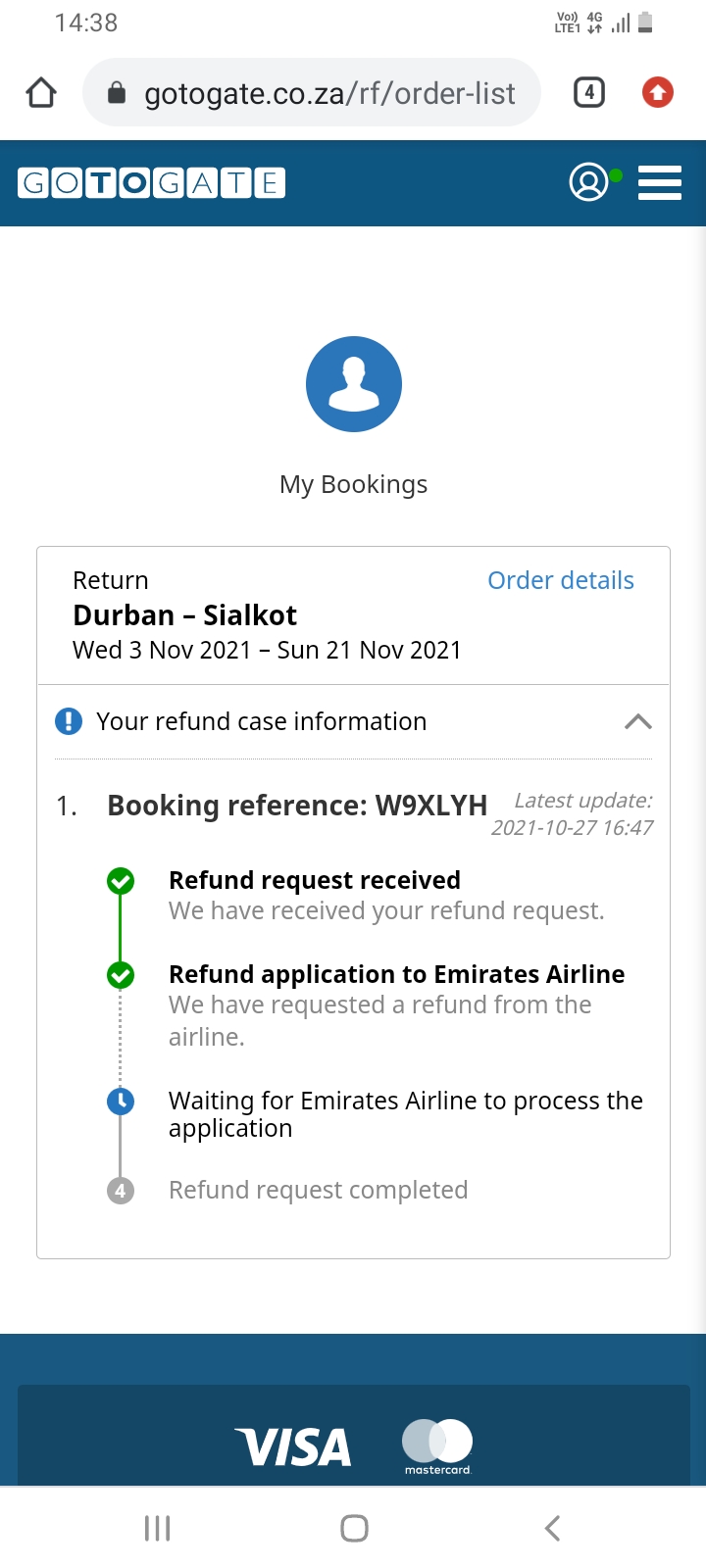The image predominantly features white and blue colors and appears to be a screenshot from a mobile browser interface. At the very top, the status bar displays the current time on the left, while the right side shows a network icon indicating 4G connectivity and a battery symbol. Below the status bar is the browser header with a home icon on the left side and a URL in the center that reads "goto gate.co.za/RF/otherlist."

Directly beneath the URL, the "Go to Gate" logo is prominently displayed. The main content area showcases a section titled "My Bookings," which includes a profile icon. Within this section, additional options like "Return" and other details are visible. 

Central to the image is the flight information, indicating a journey from Dubai to Seattle scheduled from Wednesday, November 17th, 2021, to Sunday, November 21st, 2021. An area of the image labeled "Your Refund Case Information" provides the booking reference code: W9XLYH.